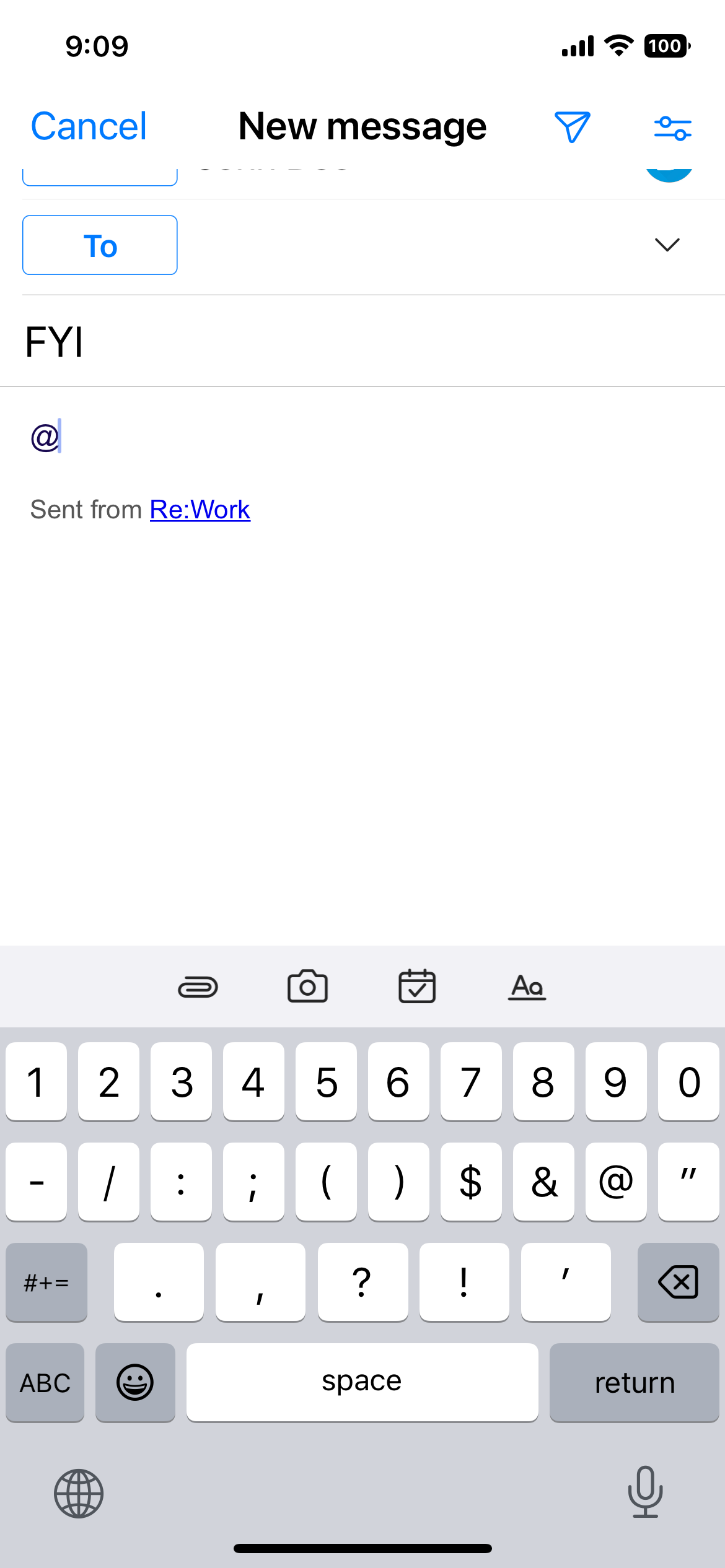The image displays an email application interface for composing a new message. At the top center of the screen, the title "New Message" is prominently displayed in black text. To the left of the title, a "Cancel" button is positioned, written in blue, allowing the user to discard the email draft. To the right of "New Message," there is a "Send" button, also in blue, indicating the option to send the completed email.

On the top right corner of the screen, a blue settings icon, likely for notifications or additional options, is visible. Below the "Cancel" button, there is a "To" field marked by blue text, where the user can enter the recipient's email address. A drop-down menu next to this field suggests that saved recipients can be selected from a list.

The subject line below the "To" field is labeled "FYI" indicating the message is "For Your Information" and is written in black. The main body of the email contains the text "add," positioned as a placeholder for the user to input the actual message content. Directly beneath this, an automated signature "Sends from rework" is displayed, with "Sends from" in black and "rework" in blue, suggesting that it is a reply related to work.

Occupying the bottom portion of the image is a smartphone keyboard with white keycaps and black characters, indicating numbers and letters. Above the keyboard, several functional buttons are present, including options for media, camera, events or dates, and font type. The background of the entire interface is white, giving the screen a clean and minimalist appearance.